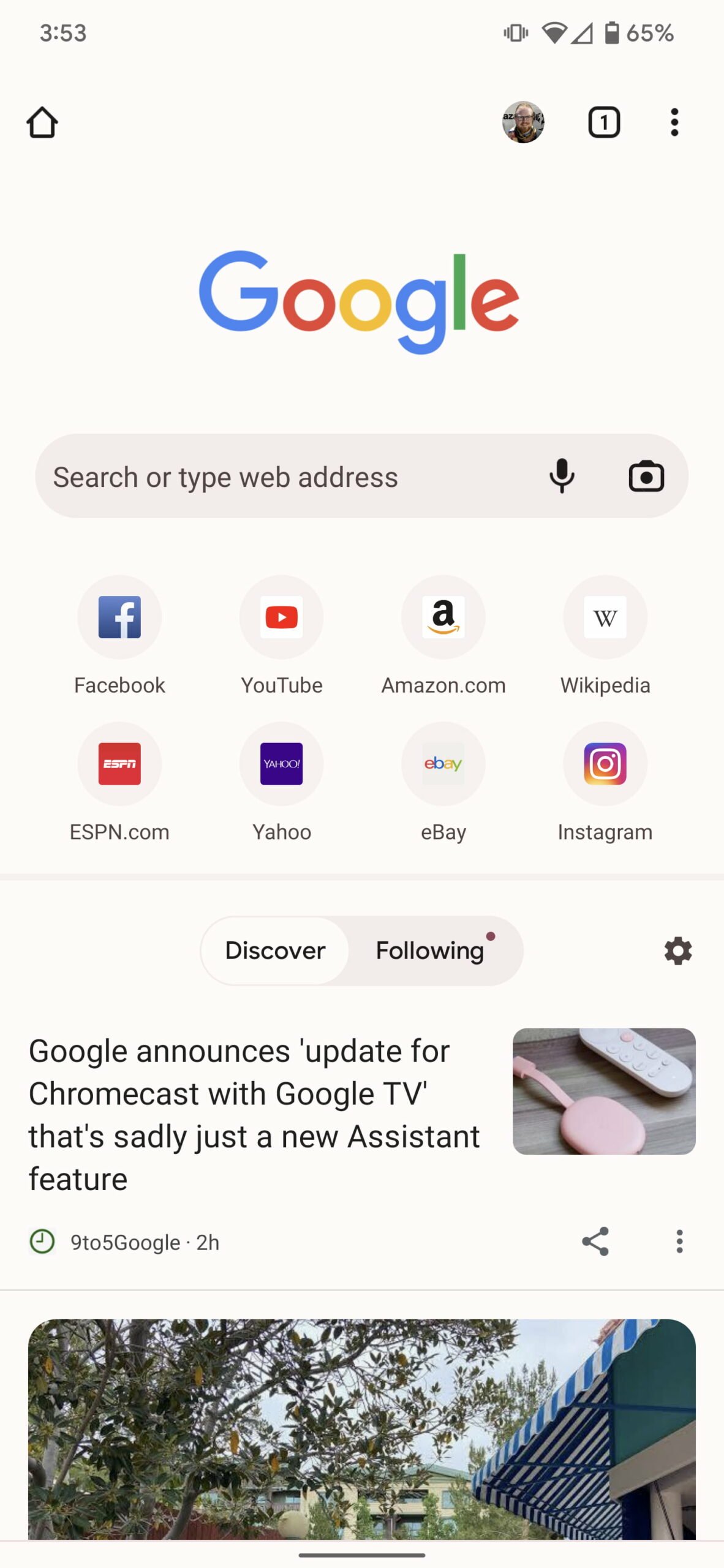The screenshot displays the home screen of a smartphone with a light beige to off-white background. In the top left corner, the black text indicates the time as 3:53. Directly below the time, there is a black outlined home symbol. To the right, the phone's status bar shows a gray vibrating icon, suggesting the phone is set to vibrate mode. The Wi-Fi signal icon is mostly gray, indicating a strong Wi-Fi connection, and the battery level is at 65%.

On the top right, there is a small profile image of the user, showing a person with a reddish beard and mustache and wearing glasses. Adjacent to the profile image is a black outlined box containing the number '1', followed by three black dots.

Centrally located is the Google logo spelled out with the letters in their respective colors: a blue 'G', a red 'o', a yellow 'o', a blue 'g', a green 'l', and a red 'e'. Beneath the logo is a gray oval with the text "social type web address" in black, accompanied by a black microphone icon and a black camera icon.

The screen also includes a grid of app icons on a light gray background. The first row consists of Facebook, YouTube, Amazon.com, and Wikipedia. The second row contains apps for ESPN.com, Yahoo, eBay, and Instagram. At the bottom of the screen, there is a notification stating: "Google announces update for Chromecast with Google TV. New assistant feature added."

This detailed depiction captures every element visible on the smartphone's home screen, providing a comprehensive view of the user's interface.